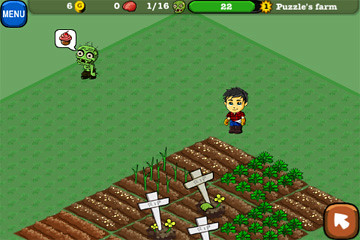This image appears to be a screenshot from an older style video game, possibly a farming simulator with some unique twists. The central scene features a garden patch with various plants at different growth stages, and notably, three crosses, which might suggest grave sites within the garden. A character stands at one corner of the garden while an alien-like creature nearby has a speech bubble saying "cupcake." Interface elements include a white arrow button in the bottom right and a blue square "menu" button in the top left. At the top of the screen, there's a yellow coin icon with the number 6, a red shape resembling a brain or heart with a 0 count, a zombie head with "1 out of 16" indicating a goal of defeating zombies, and a green bar reading 22. To the right, it says "Puzzles Farm," hinting that the game involves solving puzzles related to farming and zombies.